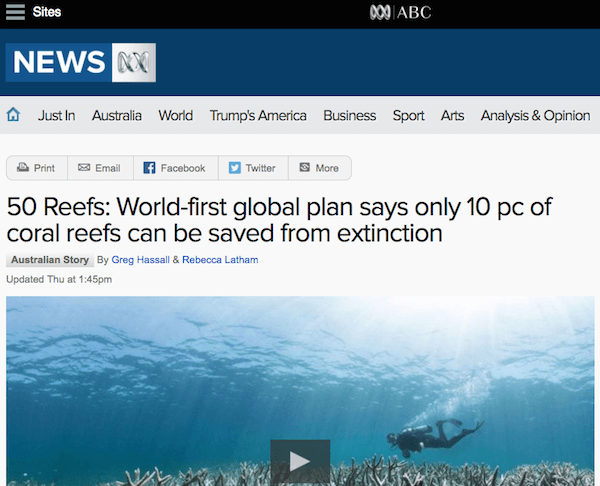This image captures the layout of a news website. At the top of the page, there is a navigation bar featuring three components: a hamburger menu, a section for various sites, and an "ABC" logo. Below this bar is the main "News" heading, followed by a series of tabs which include: Home, Just In, Australia, World, Trump's America, Business, Sport, Arts, Analysts, and Opinion. Directly beneath these tabs, there is a utility box offering options to print the page, email it, or share it on Facebook, Twitter, and other platforms.

The article title displayed is "50 Reefs: World First Global Plan Says Only 10 Pieces of Coral Reefs Can Be Saved from Extinction." The byline credits the story to Australian Story's Greg Hassile and Rebecca Latham, with an update timestamped Thursday at 1:45 PM.

Embedded within the article is a video feature showing an underwater scene. The video still captures a scuba diver who has seemingly just entered the water and is descending towards a coral reef. Sunlight penetrates the surface, casting visible rays that extend down to the reef. The video is ready to be played, as indicated by a button centered over the image.